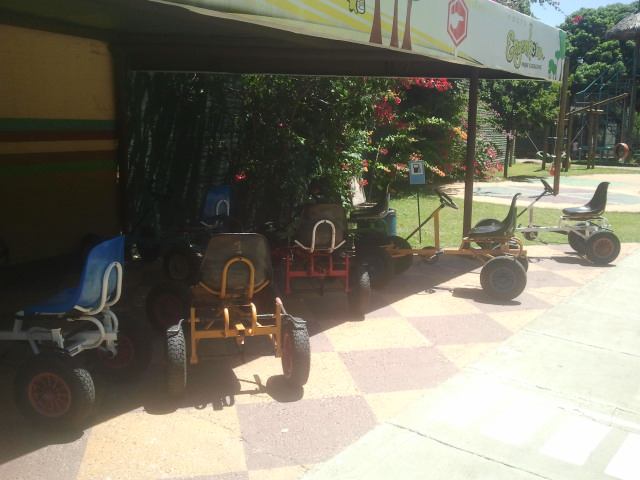The image captures a sunny outdoor scene at what seems to be a retail or garden business. Underneath a large canopy, several simple go-karts are neatly lined up, mostly in the shade. Each go-kart has four connected wheels and a seat positioned between the back two wheels, with a steering rod connecting to the front wheels. In total, there are seven go-karts, each distinctly colored: one with a green seat and green wheel, another with a yellow frame and black wheel, one with a red frame and black seat, another with a yellow frame and black seat, and two with white frames, blue seats, and red details. The background reveals a wooded area and hints at a vineyard with red flowers. Partially visible in the distance is a blurred playground, adding to the picturesque setting.